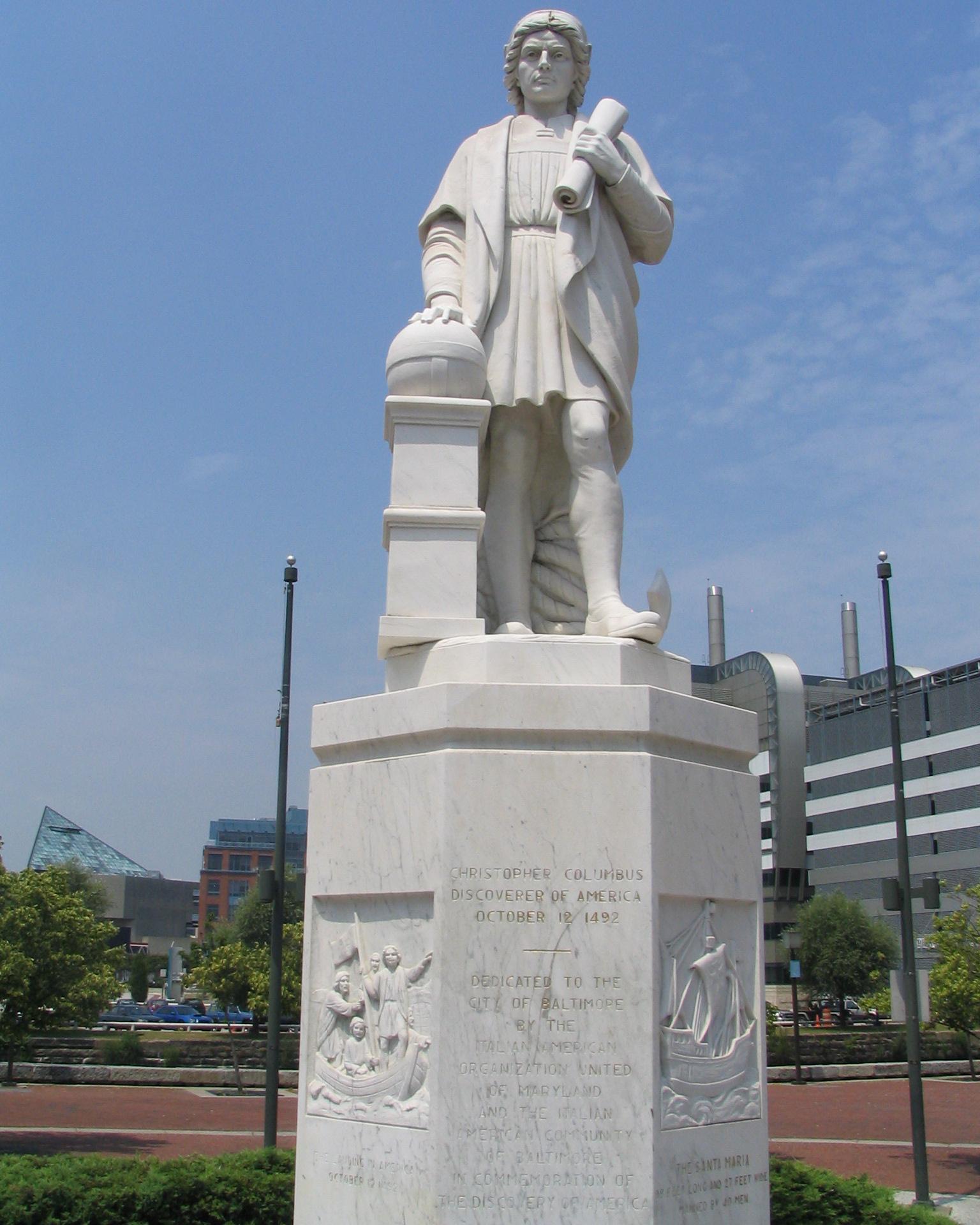The image depicts an outdoor setting featuring a grand statue of Christopher Columbus, prominently displayed atop a tall, white pedestal. The statue, crafted in white, depicts Columbus adorned in a short tunic and a cloak, holding a scroll in his left hand near his chest. His right hand rests on what appears to be a globe atop the pedestal. The pedestal is inscribed with several details: at the forefront, it reads "Christopher Columbus, Discoverer of America, October 12th, 1492." Below this dedication, the inscription becomes less legible but includes partial phrases such as "dedicated to the city of Baltimore by the...(organisation united of Maryland and the Italian) community. At the base, the words "the discovery of America" are faintly visible.

Flanking the central inscription, the pedestal features detailed carvings. On the left side, a scene depicts people in a boat at sea, while the right side illustrates a large, unmanned boat. The platform supporting the statue appears hexagonal, showcasing multiple engraved surfaces. The background reveals a bright blue sky with scattered clouds, red-colored pavement, and distant buildings, contributing to the outdoor ambiance of the scene.